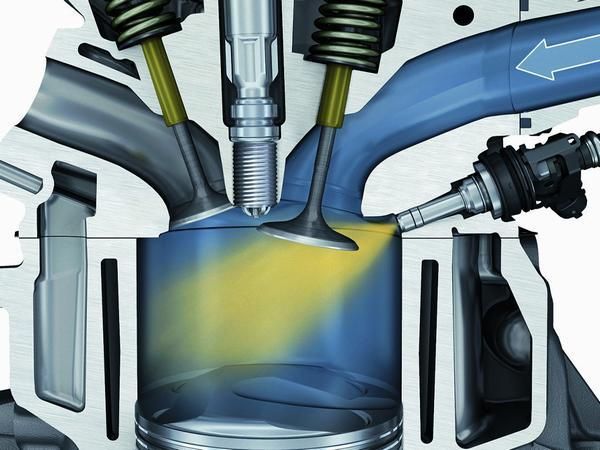The image is a detailed digital graphic, possibly illustrating the inner workings of a machine such as an engine or a complex apparatus. Central to the composition is a cylindrical glass or plastic container where various processes are taking place. Emerging from the top right of the container, there are multiple tubes and pipes, including a prominent black pipe on the left and a blue pipe on the right, which guide different substances into the chamber.

At the top, two pistons and a couple of suction-cup-like mechanisms descend from the ceiling, each connected by springs. In the middle at the top, a large screw secures the entire setup to an unseen structure. Additionally, there are blue arrows indicating the flow direction of a gas or liquid into the container, suggesting the dynamic process occurring within. On the right side, a part resembling a fuel injector shoots what appears to be yellow gas or liquid into the chamber. Accompanying the intricate machinery is a simple white background, emphasizing the device's complexity. The style and layout hint that this image might have been sourced from a magazine or a technical manual, aimed at explaining the functions of the depicted apparatus in a detailed manner.